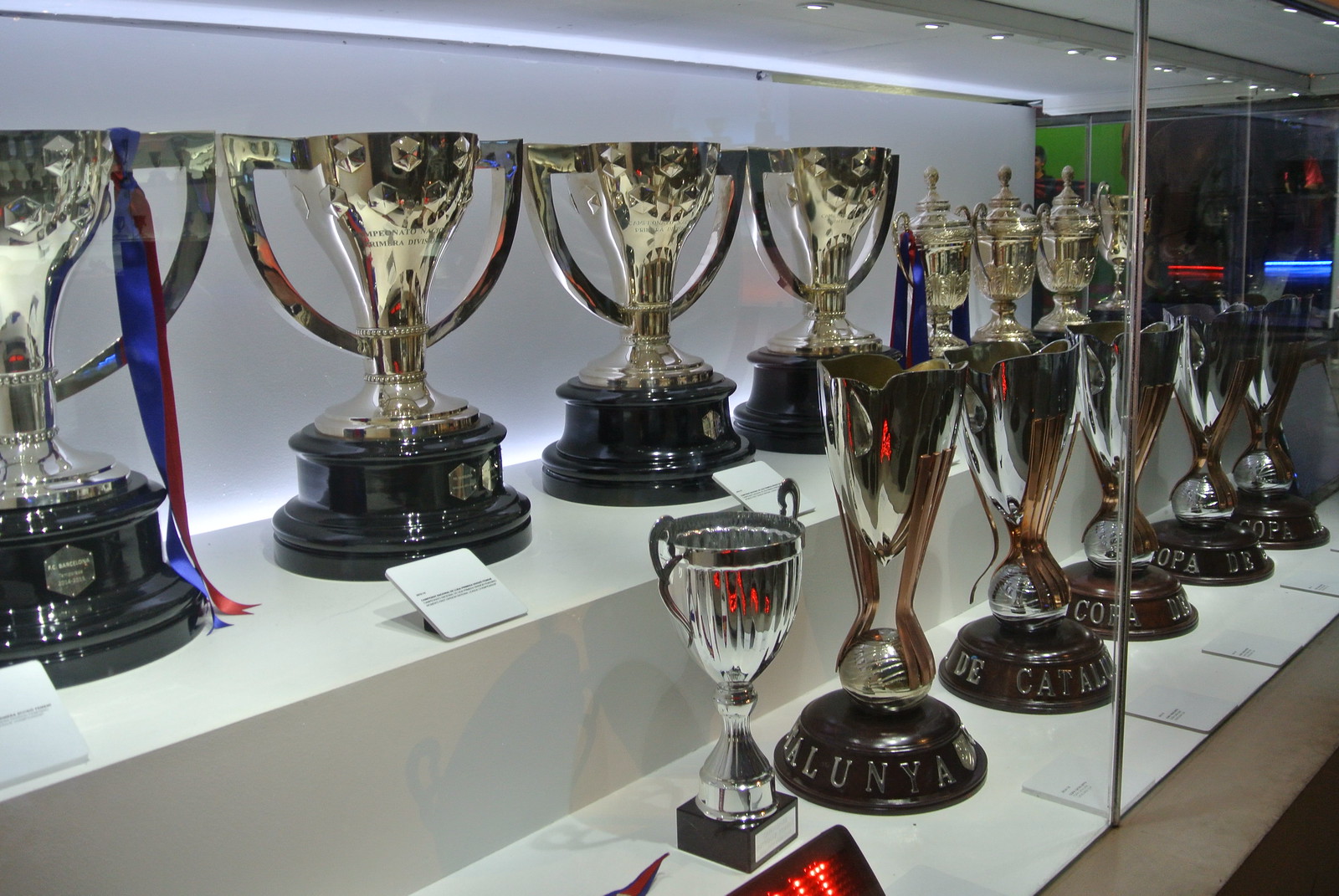The image features a large glass trophy case with a sleek, contemporary design, distinguished by white shelving and illuminated by strip lighting inside the cabinet. Positioned on two main levels—an upper shelf and a lower shelf—the case is meticulously arranged with various trophies.

On the back upper shelf, there are larger, goblet-shaped trophies adorned with handles that rest on wooden bases, each accompanied by a hexagonal plaque possibly detailing their awards and recipients. The first of these trophies has a distinctive blue and red ribbon tied to it, creating a visual highlight. Adjacent to these are smaller, equally ornate trophies shaped like cups with handles and topped with dome lids resembling crowns. At least one of these smaller trophies also features a blue and red ribbon.

The bottom shelf begins with a humble, silver trophy cup with handles. Progressing from this, there are five identical, modern-styled trophies characterized by their large, round bases with engraved letters that partially spell out "Catalunya" and "Copa," indicating a possible Spanish connection. These sleek trophies are supported by elegant stands with copper sides, each holding a tall, handle-less cup. Among these trophies, there's also a digital display panel, hinting at customizable information, though only a portion of red glowing dots is currently visible.

Through the glass of the case, a red and blue light can be seen in the background, casting a subtle glow that accentuates the trophies. The case is partially backed by a green poster depicting a person, adding another layer of visual interest to the scene. The trophies, with their meticulously detailed designs and strategic placement, reflect a significant sense of accomplishment and prestige.